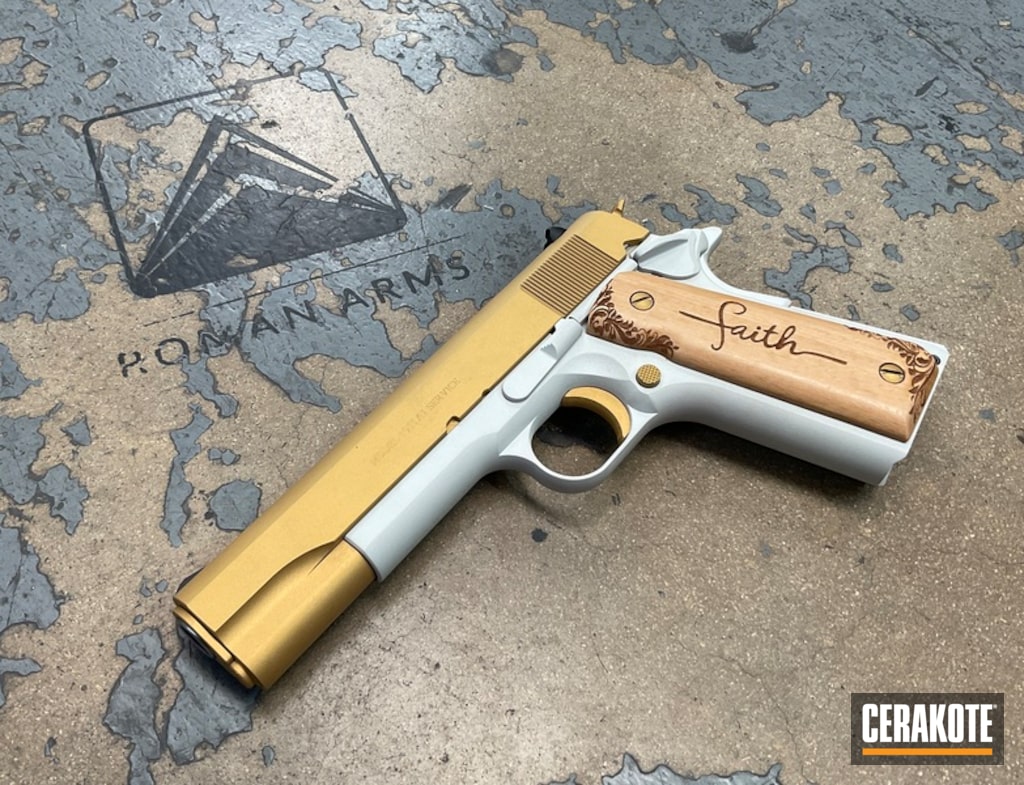The photograph captures a detailed overhead view of a semi-automatic handgun, closely resembling a classic Colt 1911, positioned on a worn, painted concrete surface. The prominent centerpiece of the image, the handgun, lies with its barrel pointing towards the bottom left corner. The weapon features a distinctive two-tone design: the lower frame, grip, and trigger guard are constructed from a white metal, while the upper slide, trigger, and safety are fashioned from a brass or gold metal. Showcasing exquisite craftsmanship, the wooden grip is intricately carved with floral patterns and bears the word "Faith" engraved into it, likely through a wood-burning technique.

The background is characterized by concrete with significant wear, revealing patches of what was once navy blue paint. Positioned to the top left of the handgun, there's a black triangular logo with the text "Roman Arms" painted beneath it, suggesting a manufacturer or a brand association. In the bottom right corner, another logo appears, consisting of a gray square with white text underlined by an orange line, spelling out "Cerakote." This setting emphasizes both the artistic and functional aspects of the firearm, presenting a juxtaposition of vintage elegance against an industrial backdrop.